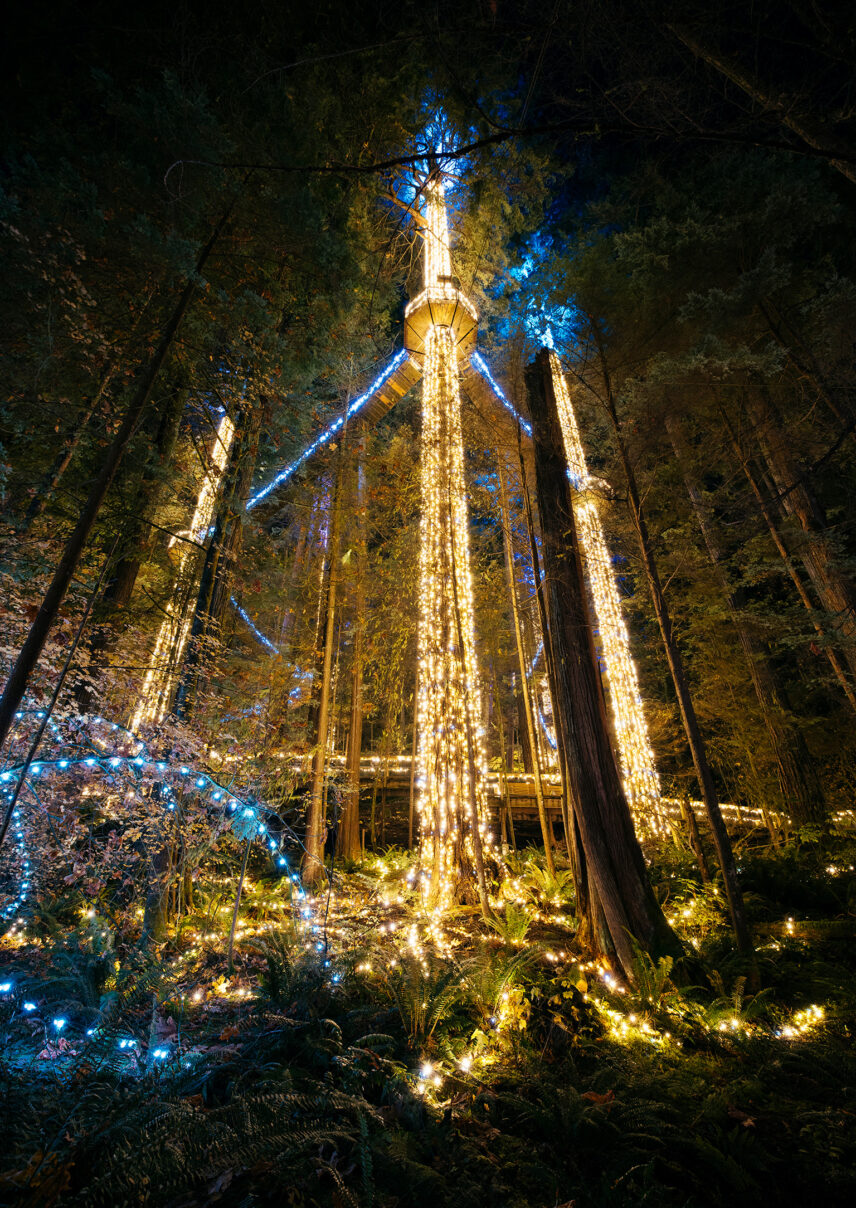This color photograph, captured in portrait mode during nighttime in a forest, showcases a striking scene of tall and slender pine trees. The trees, illuminated against the darkness, have their lower sections bare while their greenery begins higher up. Dominating the center is a tall tree, wrapped meticulously with vertical strands of gold and white lights, creating a shimmering effect. About three-quarters up this tree, a circular platform is adorned with more golden lights, and at its pinnacle, blue lights glow vividly.

Accompanying this centerpiece are two additional trees in the background, similarly decorated, though their details are less discernible due to their positioning further away. Connecting these illuminated trees is a strand of blue lights, enhancing the ethereal ambiance.

At the bottom left-hand corner of the image, strands of blue lights lay spiraled and bunched up on the forest floor, interspersed with piles of white light strands resting on the green foliage. The silhouetted shapes of other trees loom softly in the background, adding depth to this magical woodland scene.